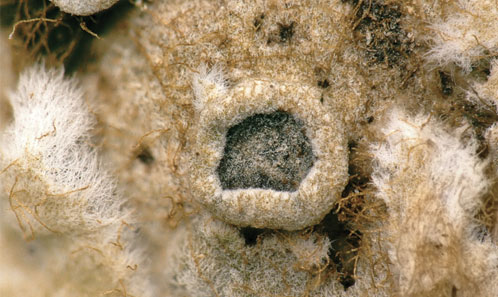The image depicts a detailed close-up, resembling a bird's nest-like structure at its center. This focal point is a round, soft circle composed of a mix of tannish, white, and brown hair-like or stringy materials, interspersed with darker areas and a few black dots. The nest-like structure is surrounded by light-colored, puffy objects intertwined with thin, brown twig-like elements. The depth of field blurs the perimeter, making the central object appear more prominent and sharply focused. Despite the organic and slightly ambiguous nature of the subject, the intricate texture and color variations suggest it might be a macro shot, possibly of fur or a plant.